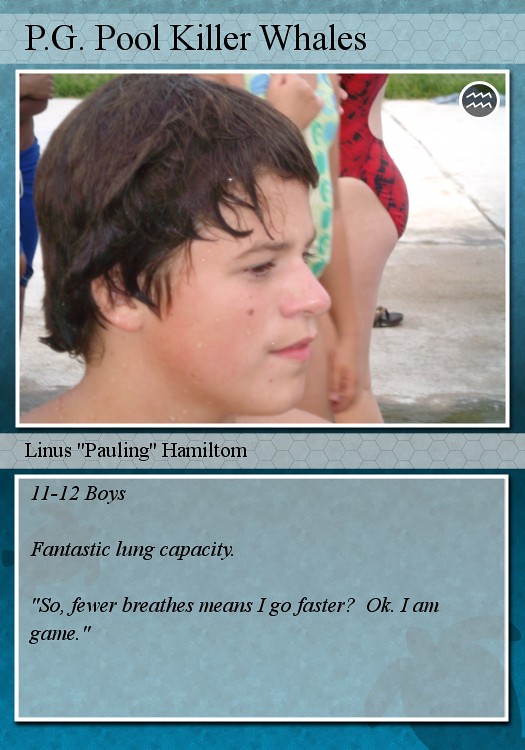The image is a visually striking trading card with a greenish-blue background, prominently labeled "PG Pool Killer Whales" at the top in black text. Central to the card is a close-up, side-profile photograph of a young boy with wet, shaggy dark brown hair, and pale skin, looking to the left. Behind him, the wet cement poolside and the side profiles of two girls in one-piece swimsuits—one red and the other greenish-blue—are visible, suggesting a swimming pool setting. Middle of the card features the name "Linus Pauling Hamilton," followed by the details "11-12 Boys," highlighting his "Fantastic Lung Capacity." This is further emphasized with a motivational quote in black text: "So fewer breaths means I go faster. Okay, I am game."